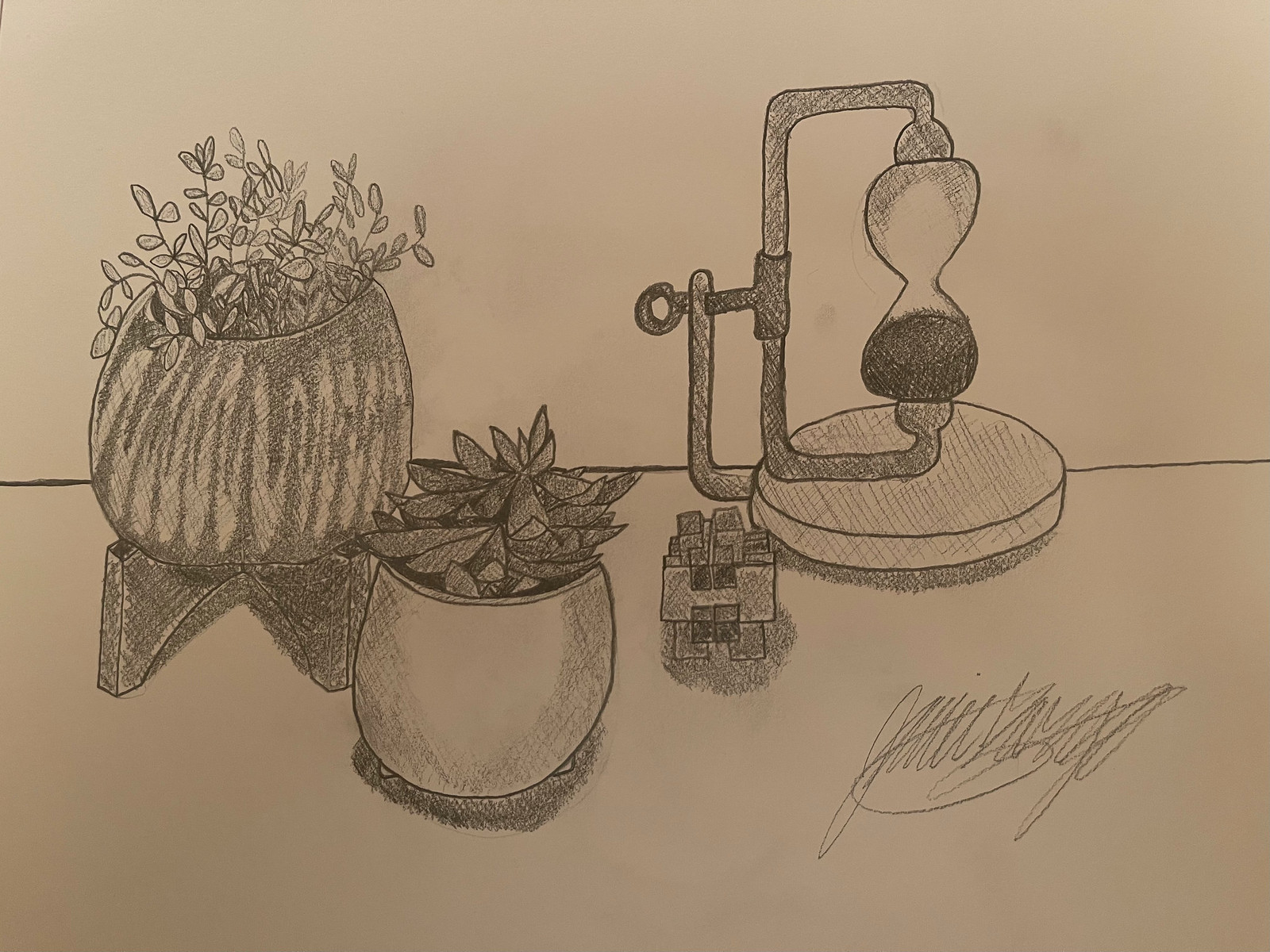This detailed pencil drawing, possibly from a high school class, features four distinct objects, meticulously shaded with techniques such as cross-hatching. On the left is a potted plant with small leaves, housed in a pot with a wavy design, standing on a wooden planter stand. Adjacent to it, and slightly in front, is a shorter potted plant with larger, darker flowers, exuding a traditional appearance. Between these plants sits a mysterious, cube-like object whose purpose is unclear. On the right side of the image, a unique hourglass is captured, seemingly held vertically within a vice-like structure that resembles a handle of a hacksaw, supported by a metal frame atop a wooden base. The artist’s elaborate signature is prominently displayed at the bottom right corner of the large sketchpad drawing, adding a personal touch to the composition.